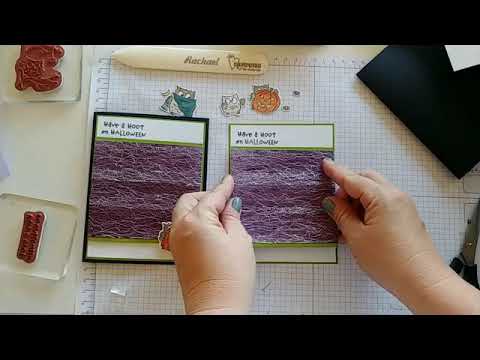In this top-down photograph, a person with green-painted fingernails is engaged in a detailed scrapbook project on a white, grid-marked measuring mat. The mat features black markings and units along the top and left sides. On the left side of the mat, there are two upturned rubber stamps in clear mounts. Across the top of the mat are Halloween-themed stickers, including a jack-o'-lantern and two monster figures, as well as a white stick inscribed with the name "Rachel" in script.

The workspace contains two greeting card panels placed centrally on the mat; the left panel has a green border, a black text at the top, and a purple straw-like fabric square in the center, while the right panel has a similar layout, with hands positioning another purple fabric square onto it. Scissors, construction paper, and an assortment of arts and crafts supplies are scattered around the workspace, contributing to the creative Halloween-themed scene.